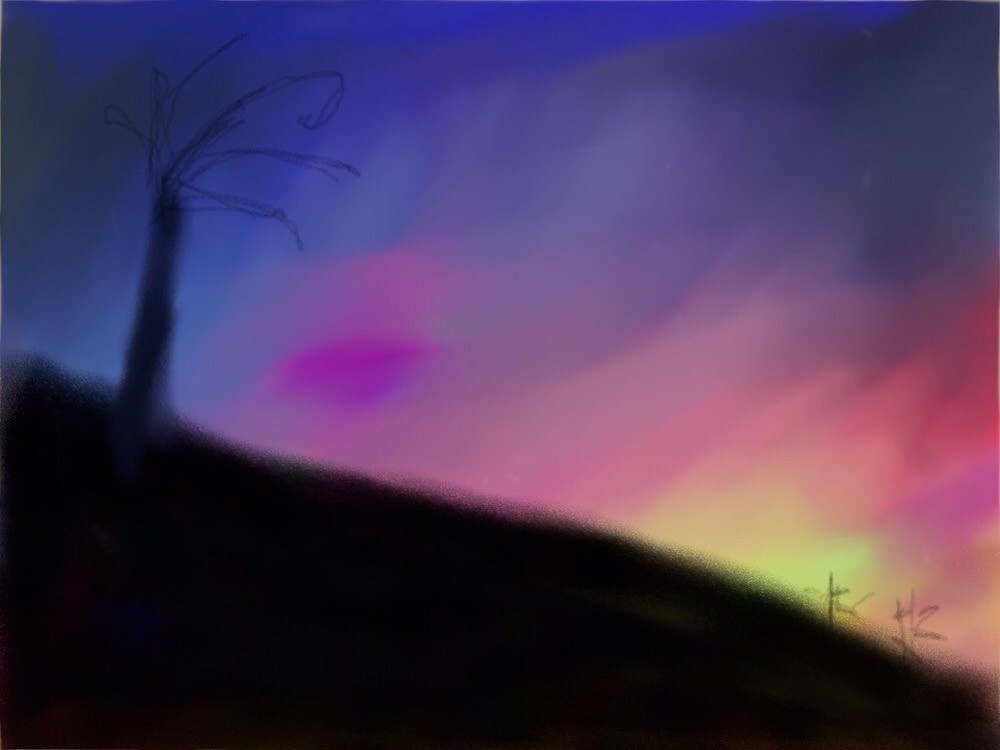This striking illustration, resembling a painting on canvas, depicts a mesmerizing sunset sky transitioning through a spectrum of colors. On the left-hand side, the sky starts in deep blue and black hues, gradually shifting through varieties of blue, then purplish-gray, seamlessly blending into dark and light pinks. Moving towards the right, the colors transform into vibrant yellow, coral, magenta, red, and orange shades, creating a beautiful, blended backdrop.

In the foreground, a jet black hill extends diagonally from the bottom right corner to the center left of the image. The hill, appearing larger on the left and narrowing towards the right, is adorned with scribble-like plants at its base on the lower right. Perched on the top left of the hill is a stark black tree. The tree features thin, squiggly branches emanating from its trunk, simulating the form of leafless branches. This meticulously detailed and colorful artwork captures the eye with its rich hues and striking silhouettes, creating an overall harmonious and enchanting scene.